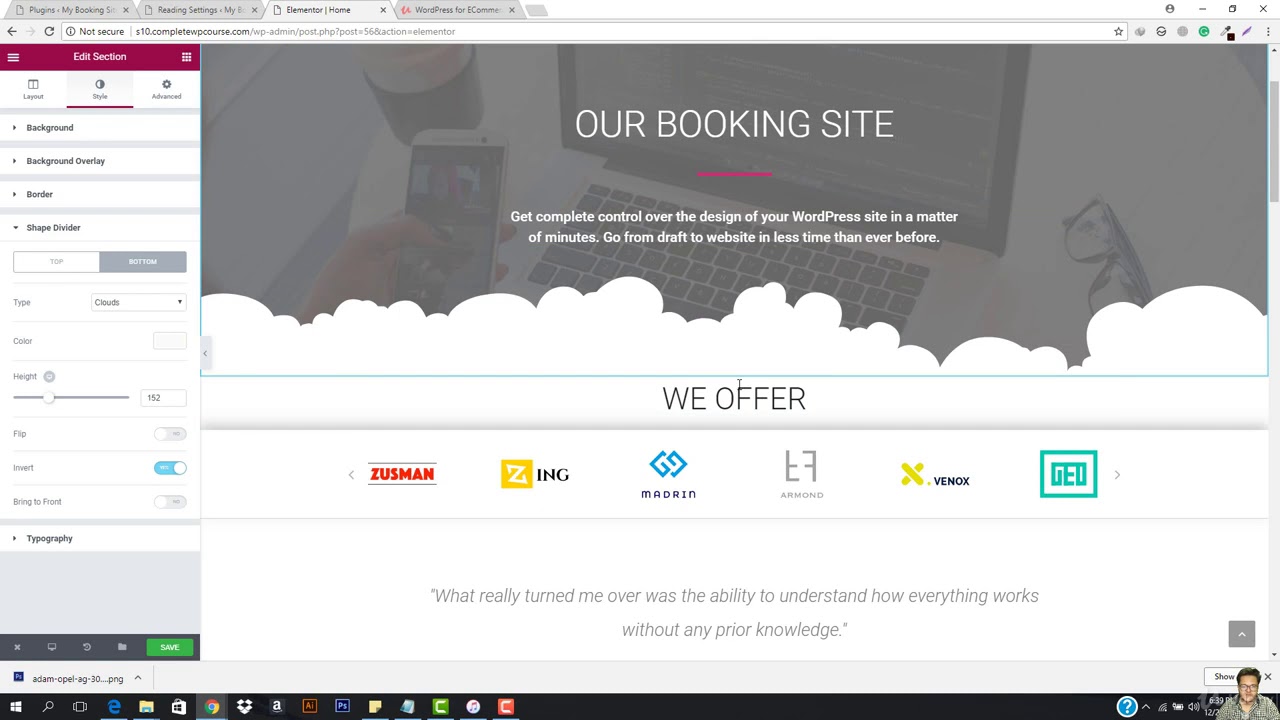A screenshot of a booking website displaying the third of four open tabs. The user's navigation bar is located on the left side of the screen, featuring a small hamburger menu icon at the top left. Adjacent to this, a square grid with dots can be seen. A prominent purple header reads "Edit Section" at the top of the left-hand navigation bar. Underneath the header, the available options are "Layout," "Style," and "Advanced." The current selection is on the "Style" page, revealing various customization options: "Background," "Background Overlay," "Border," and "Shape Divider." For the Shape Divider, there are several controls including toggles for different buttons, and settings for type, color, height, flipping, inverting, positioning at the foot, and typography. All these options are neatly listed in the left-hand navigation bar for the user to adjust.